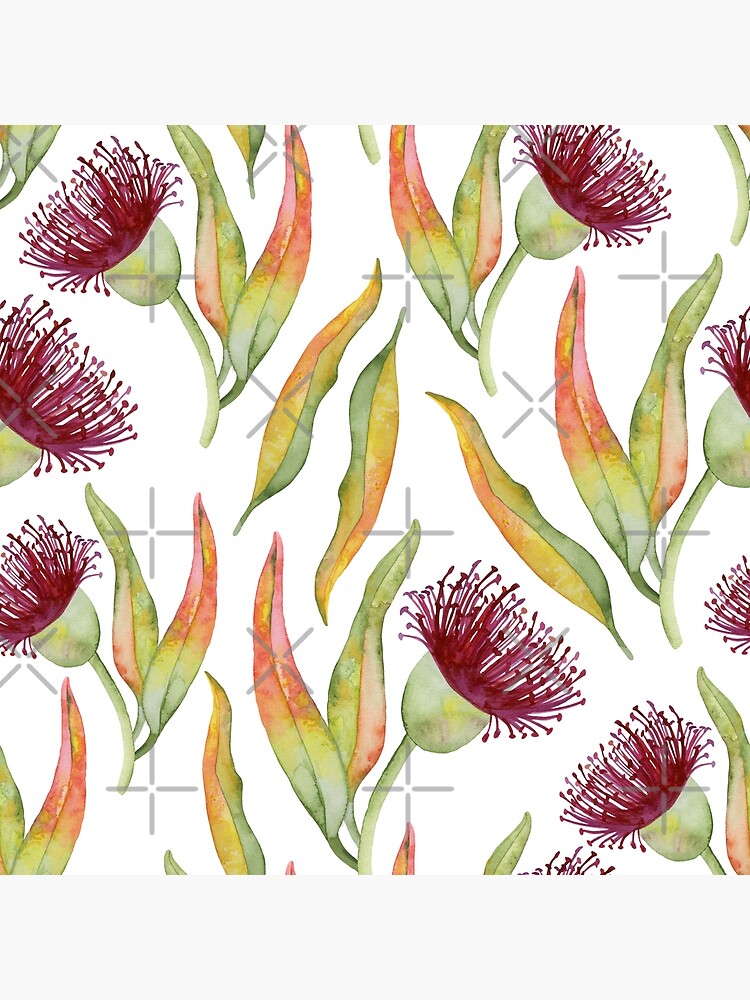The image showcases a patterned art print that resembles wallpaper with a cream or white background. It features long, thin leaves that are orange, yellow, and green, described as pod-like, with alternating green stems. These stems support unique flower buds that are pale green and bell-shaped, covered densely with maroon filaments ending in solid maroon tips. The floral arrangement is intricate and features at least some flowers potentially dark green or pink. The background is overlaid with gray X's and plus signs, potentially as a watermark, adding to the patterned complexity. There are rectangular gray shapes at the top and bottom of the image. The entire composition appears almost embroidered due to its detailed and textured appearance.